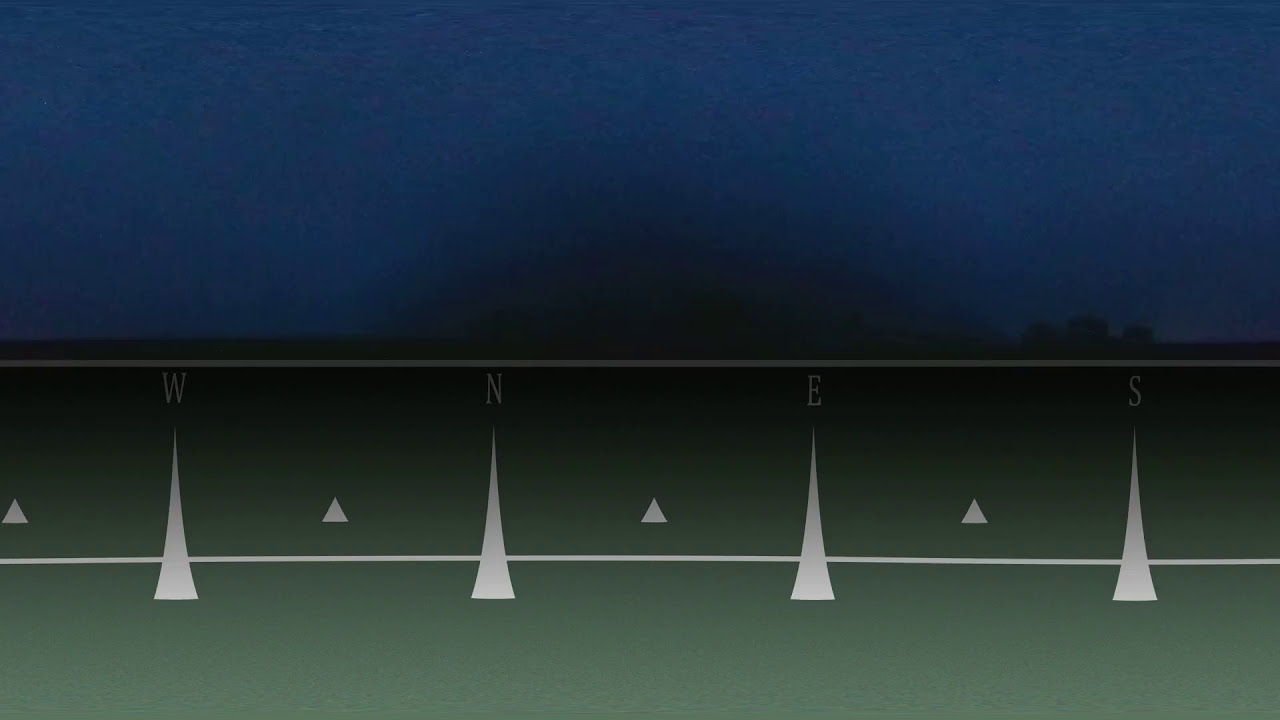In the photograph, a dark green surface stretches into the distance, bisected by a prominent white line running down the middle. Arranged along this line are a series of white cones, with four larger cones interspersed with smaller ones. Each of the larger cones is clearly labeled with the letters W, N, E, and S for West, North, East, and South, resembling a stretched-out compass. Two white lines cross the image: one runs along the bottom, about two-thirds down the height of the large cones, while the other sits above the cones, parallel to the first. The foreground area appears marked with these white or light gray shapes against the green background. The sky, a gradient of blue transitioning into deeper shades, spans the upper portion of the image, occasionally interrupted by hazy trees or blurred outlines of buildings, giving an overall grainy and smoky appearance.